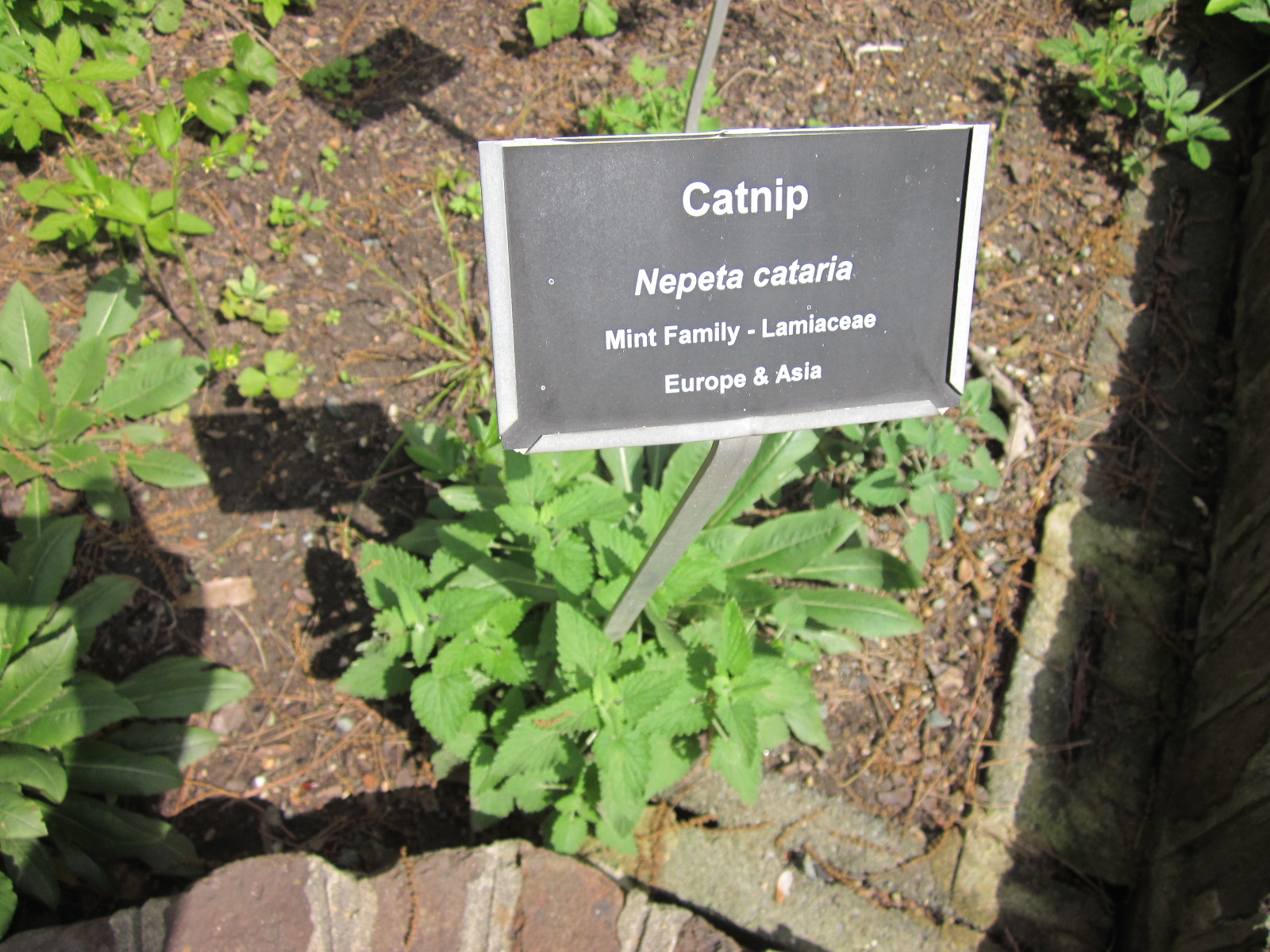In the center of the image, a catnip plant, scientifically known as Nepeta cataria, stands prominently highlighted among a variety of other plants in a backyard plantation. The catnip is identified by a sleek rectangular black sign with white text that provides detailed information about the plant. The sign reads: "Catnip, Nepeta cataria. From the mint family, Lamiaceae. Native to Europe and Asia." This detailed sign adds an informative touch to the lush greenery, making it easy to identify the catnip in the midst of the diverse botanical collection. The background surrounding the catnip is filled with a mixture of different plants, creating a vibrant and rich natural tapestry.